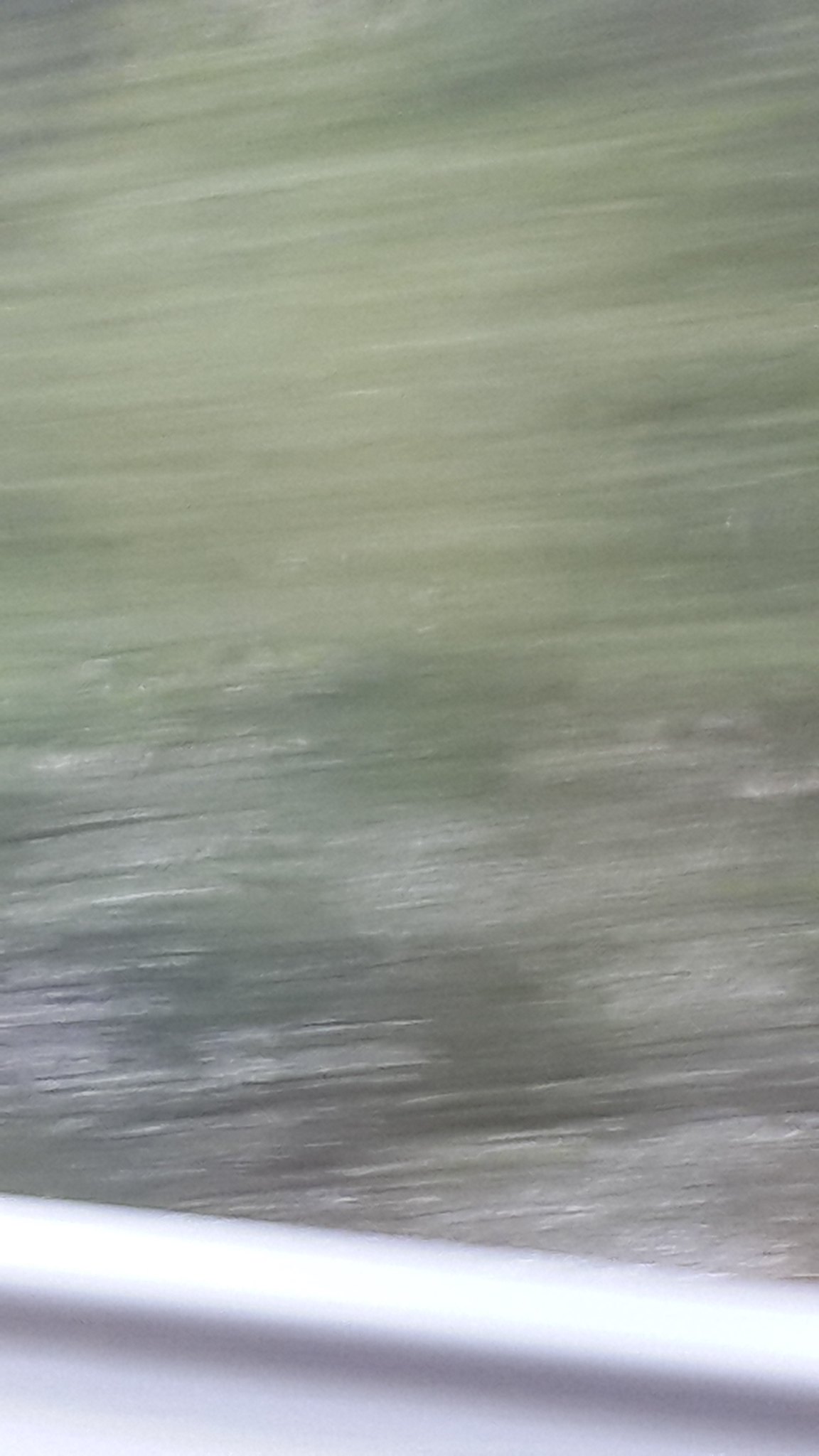This vertically-oriented, rectangular image captures a blurred, dynamic scene. At the bottom, a silver guardrail, illuminated by sunlight on its upper surface while shadowed beneath, suggests the speed of a vehicle moving down a highway. This guardrail stretches across the width of the image, contrasting with the blurred backdrop of greenery and gray hues. Above the guardrail, streaks of gray, green, and white blend into a striping pattern, flowing left to right, further emphasizing the motion. Dominating the top half of the image, varying shades of green, from pale to deep hunter, create a painterly effect reminiscent of light brush strokes gently sweeping across a canvas. The overall blur evokes a sense of rapid movement through a lush, green landscape.